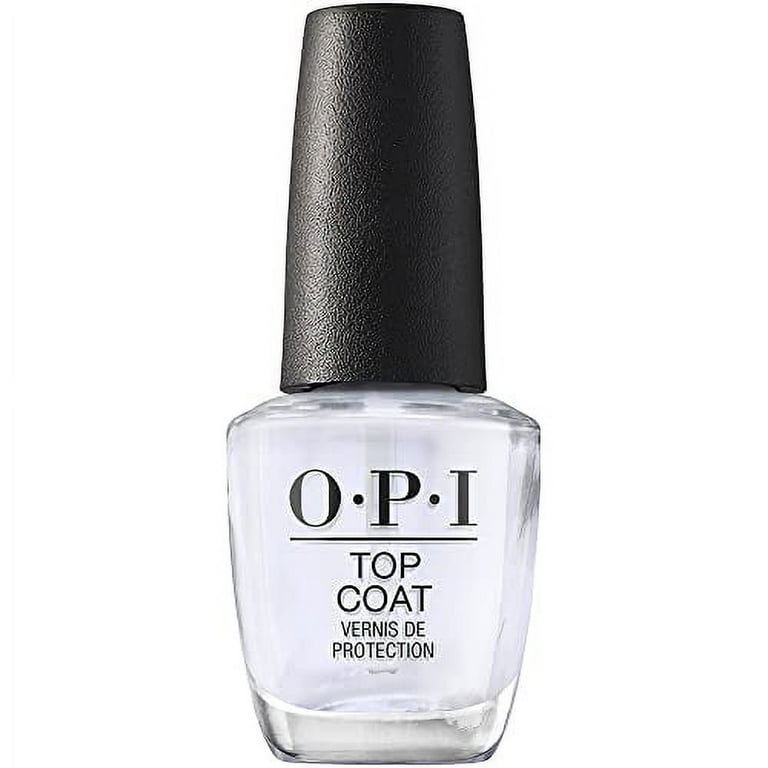This image features a close-up product photo of an OPI brand nail polish bottle, distinctly isolated against a pure white background, likely achieved by removing the original background, possibly with a green screen. The clear glass bottle has a thick base and gradually widens towards the top, with flat sides and curved edges. It is filled with a clear liquid, aligned with the typical design of nail varnish containers. The bottle has a large, long, rectangular black plastic cap that flares out slightly and is round at the top, which can be unscrewed to reveal the applicator brush inside.

The front of the bottle prominently displays the brand name "OPI" in large black capital letters, under which a horizontal black line is drawn. Beneath this line, in smaller black letters, the label reads "Top Coat" followed by "Vernis de Protection." The photograph is likely intended for promotional use by the manufacturer or for listing on an e-commerce platform. With an approximate height of three to four inches, the bottle's meticulous design and clear labeling make it unmistakably a nail polish product meant for a protective top coat application.